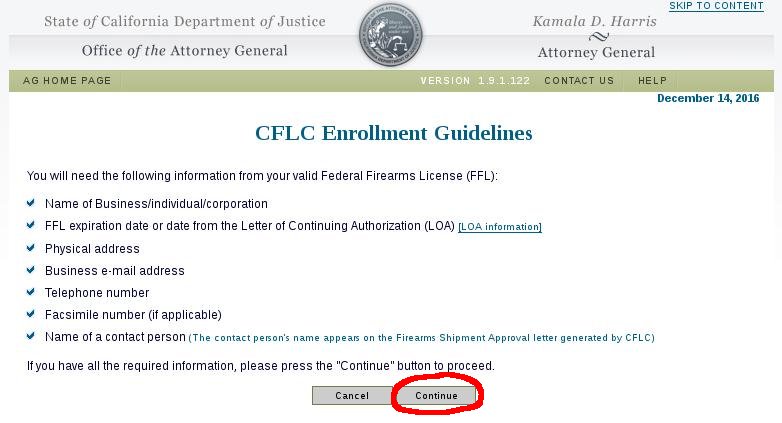This image showcases a webpage from the California Department of Justice. At the top center of the page, the official logo is prominently displayed. To the right, various administrative details are listed including Kamala D. Harris, then Attorney General, along with navigational links such as "Skip to Content," "Office of the Attorney General," and the "Attorney General Homepage." The page details version 1.9.1.122 and provides links for "Contact Us" and "Help," along with a timestamp indicating December 14th, 2016.

The main content of the webpage outlines the CFL-C Enrollment Guidelines, which stipulate the necessary information required for an application. Applicants need to provide details from a valid Federal Firearms License (FFL), including the name of the business, individual, or corporation, the FFL expiration dates, the dates from the later of continuation authorization (LOA), the physical address, business email address, telephone number, and fax email number if applicable. Additionally, the contact person's name must be included as it appears on the firearms shipment approval letter generated by CFL-C. If the user has all the needed information, they are prompted to proceed by pressing the "Continue" button, which is highlighted in red for emphasis.